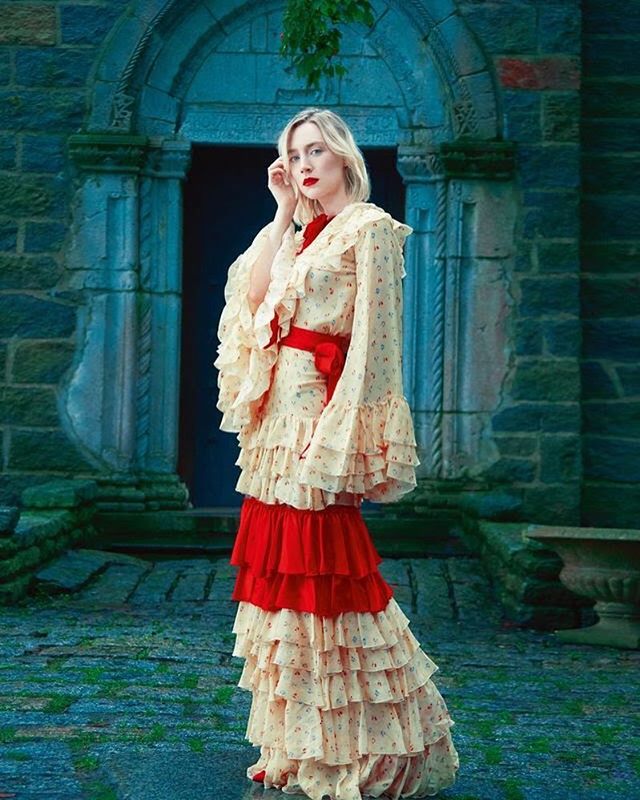In this striking image, American-born Irish actress Saoirse Ronan is depicted standing in front of an ancient-looking stone building, reminiscent of a castle entrance. The backdrop features a grand stone archway with visible patches on each side of the door, and a lush hanging plant draping down to accentuate the age-old structure. The stone cobblestone pathway beneath her feet shows signs of time, with moss sprouting between the pavers. The nuanced background includes a blend of cinder blocks and bricks in hues of blue and green, with some gray and white mortar, interspersed with patches of red brick and leafy greens hanging from above.

Saoirse Ronan stands slightly off-center toward the bottom of the image, capturing attention in a graceful and elegant pose. She wears a cream-colored gown adorned with intricate prints and a red bow around her waist. The multi-layered skirt of the gown showcases tiers of pleats, connecting the ensemble's overall refined appearance. Her right arm is raised as she gingerly touches her blonde hair. Complementing her sophisticated attire, she has bold red lipstick, and she appears to be making direct eye contact with the viewer, adding a sense of engagement.

The composition creates an overall quaint yet regal atmosphere, emphasizing the historical and lush surroundings, while highlighting Ronan's poised and captivating presence.